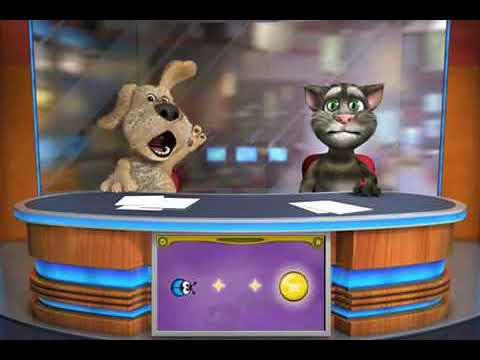In this whimsical, computer-generated image, a dog and a cat, rendered as cartoon characters, are positioned at a news desk, seemingly delivering a news segment. The dog, a tan and brown furry labradoodle, is on the left side of the image with one ear perked up, the other down, its mouth open in what appears to be an excited or assertive expression. It has its right paw on the desk and its left paw raised, as if making an emphatic point. To the dog's left, our right, sits a black, gray, and white cat with a concerned or frowny face, embodying a nervous demeanor. Both animals are seated in red chairs behind a news desk that features a blend of medium blue and brown wood with a gray top surface. In front of them lie scattered white papers, adding to the newsroom ambiance. Behind them, a large screen displays a blurred cityscape, reinforcing the studio setting. The front of the desk is adorned with a blue ladybug, stars, and a sun emblem, hinting at a playful, possibly children's show or cartoonish context.